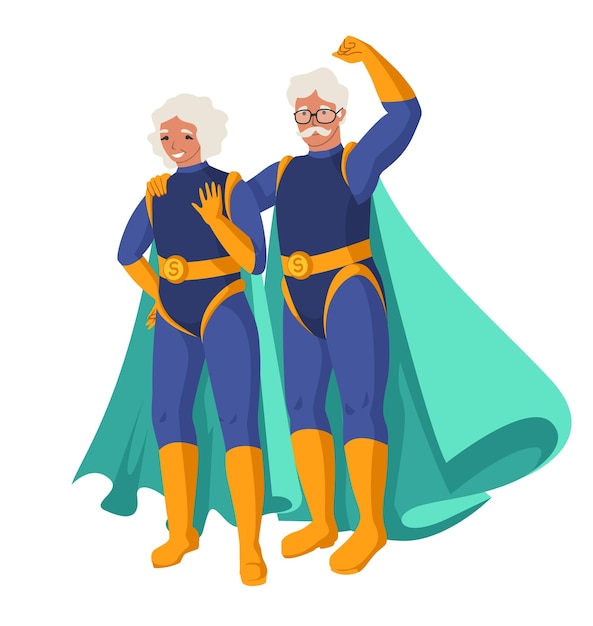This is a detailed digital illustration of two elderly superheroes, a man, and a woman, standing side by side. The man, positioned on the right, sports short gray hair, bushy gray eyebrows, a gray mustache, and black wire-framed glasses. He is shown triumphantly lifting his left fist in the air while his right hand rests on the woman's right shoulder. The woman, positioned to his left, mirrors his appearance with short gray hair and bushy eyebrows. She is smiling slightly and has her right hand placed on her hip while her left hand is raised as if waving. Both characters are adorned in matching blue bodysuits with darker blue centers, complemented by yellow boots, yellow belts featuring an "S" buckle, and light bluish-green capes draped over their shoulders. Their outfits suggest a theme of senior superheroes, possibly "Super Seniors," united in a display of strength and camaraderie.